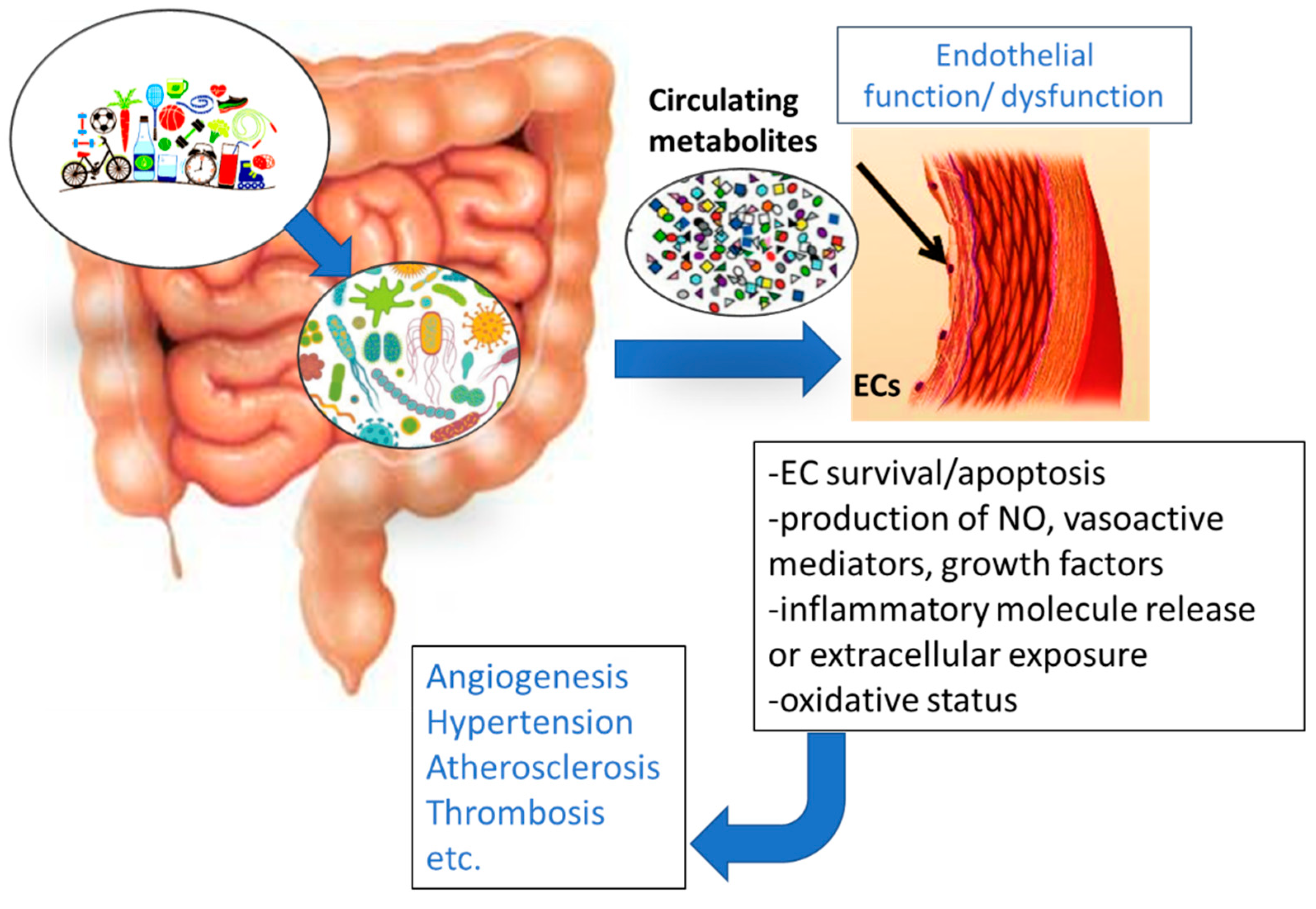The image is a detailed scientific diagram of a person's gut, focusing on the interactions within the intestinal tract and the impact of the gut microbiome. On the left side, there is a colored illustration of the small and large intestines, with a couple of ovals containing colorful microbes symbolizing the gut bacteria. An arrow labeled "circulating metabolites" points towards a section titled "endothelial function/dysfunction," which includes a depiction of reddish-orange tissue cells. Below this section, multiple physiological processes are listed, including endothelial cell survival, apoptosis, NO production, vasoactive mediators, growth factors, inflammatory molecule release, and oxidative status. Another blue arrow leads to a final box that outlines several health outcomes: angiogenesis, hypertension, atherosclerosis, and thrombosis.